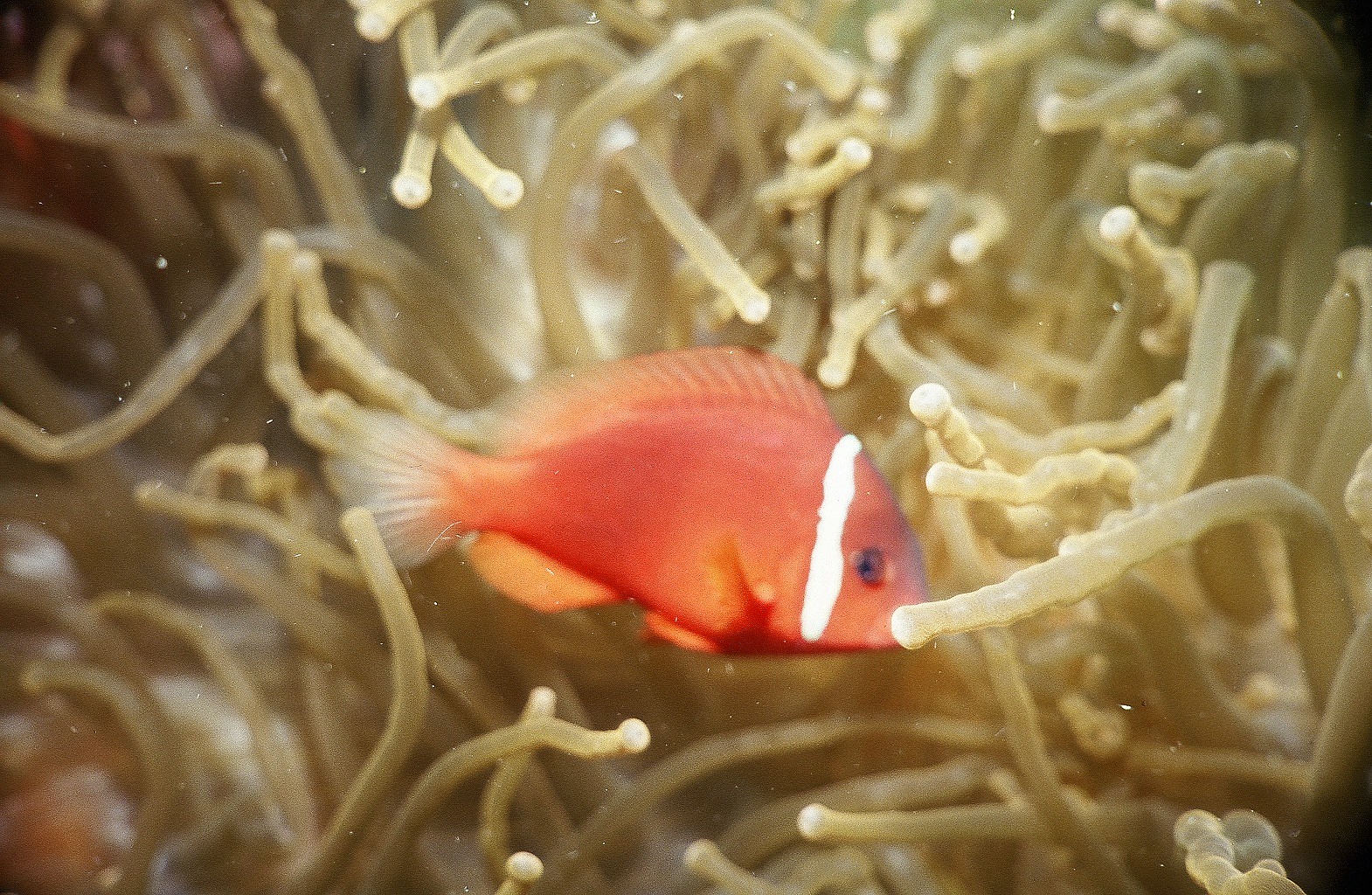This underwater image, likely taken in an aquarium, features a small, golden-orange fish centrally framed and surrounded by sea anemone-like creatures. The fish, resembling a goldfish in size, has a distinct white stripe running vertically just behind its eye and is adorned with white-tipped fins and a tail that fades from its orange body. The anemone-like structures, which evoke the appearance of long, jelly-like spaghetti strands with rounded ends, encompass the fish, creating a captivating scene with light softly filtering through the water. Tiny specks floating around add depth and detail to the watery ambiance. There might be another slightly blurred fish visible in the bottom left corner, enhancing the richness of the underwater environment.